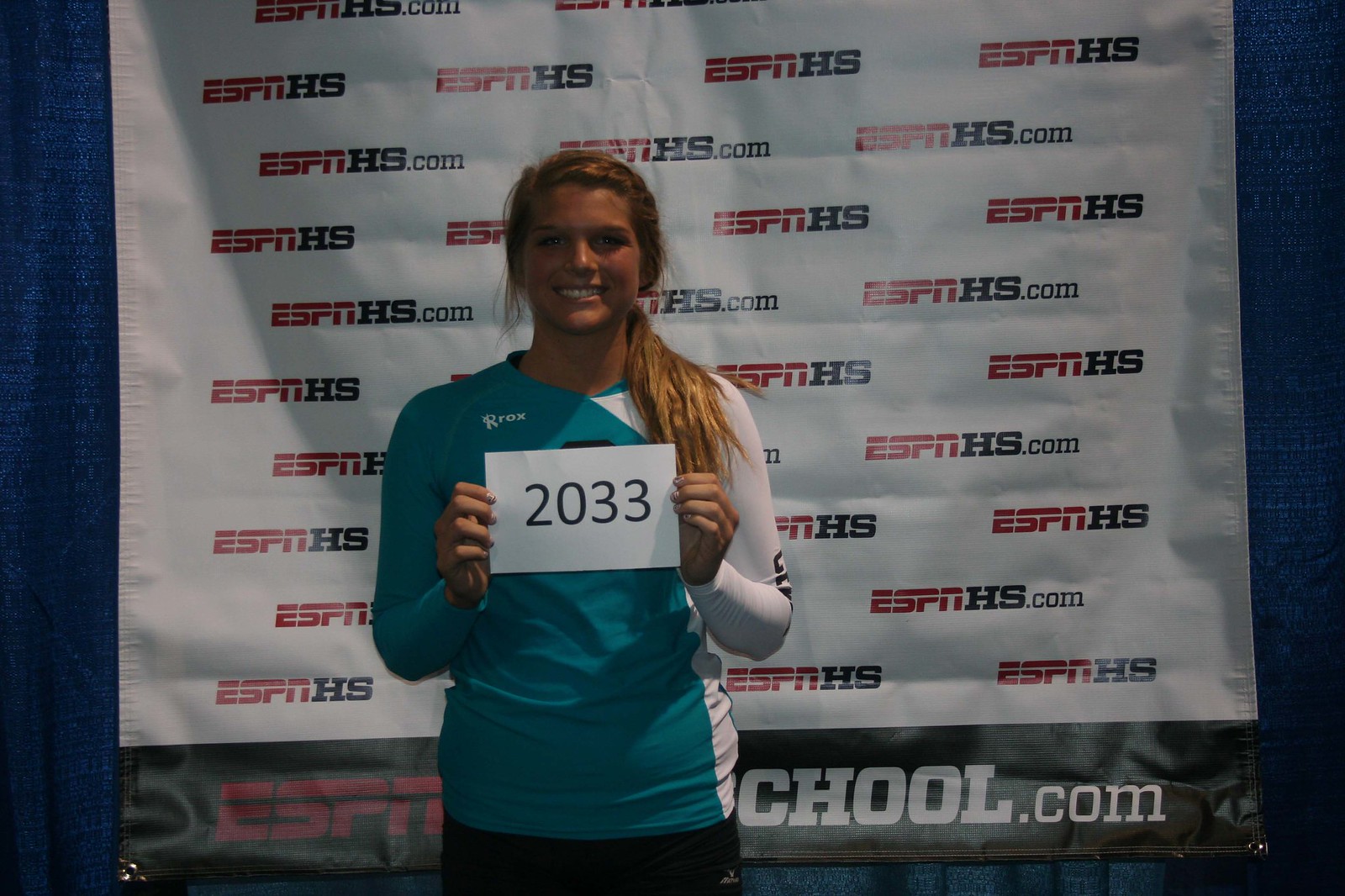The photograph captures a teenage girl, likely an athlete, standing victoriously on a podium. She has long blonde hair pulled into a ponytail, draped over her right shoulder, and a fit, athletic build with broad shoulders. She wears a distinctive uniform: a light blue shirt with a turquoise front and left sleeve, and a white section on the right sleeve and side, paired with black shorts. She is smiling and energetically holding up a white placard displaying the number "2033" in black text. Behind her, a large, square banner hangs against a blue backdrop, predominantly white with repetitive branding. The banner features "ESPN HS" and "ESPNHS.com" in red and black text, indicating the association with ESPN's high school sports coverage. The banner's bottom strip is black with the text "ESPNHighschool.com" in white. The overall scene suggests a moment of triumph and excitement within a high school sports event.